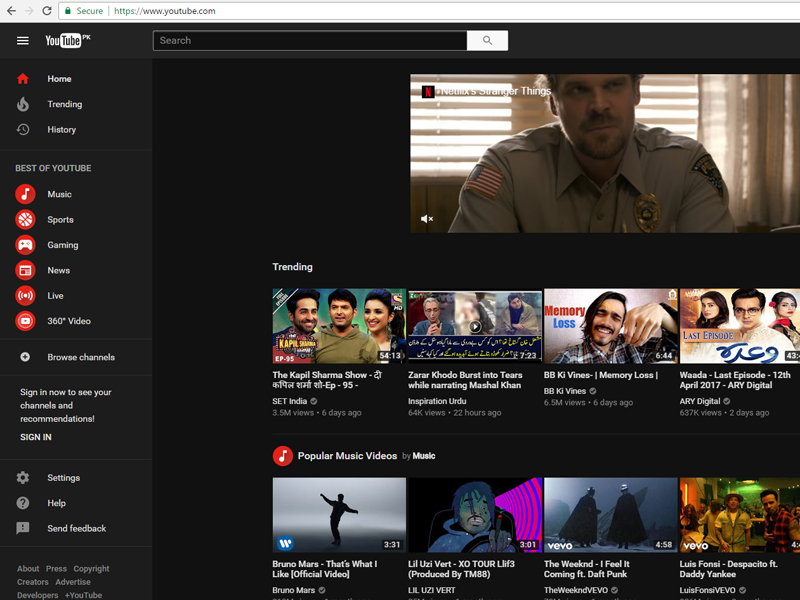The image displays a YouTube homepage interface, potentially from another country or customized to showcase content in multiple languages. The URL in the search bar reads "www.youtube.com", accompanied by a green secure logo, a back arrow, and a refresh icon in the upper left corner. A black section beneath the search bar features a white three-horizontal line icon adjacent to a YouTube icon labeled "PK", followed by a black search bar with a white search button.

On the left-hand side, there are a series of clickable options: Home, Trending, History, and a section titled "Best of YouTube" which includes categories such as Music, Sports, Gaming, News, Live, and 360 Video. Additional links include "Browse Channels" and "Sign in to see your channels and recommendations," followed by "Sign in," "Settings," "Help," and "Send Feedback."

The right-hand side displays video thumbnails featuring popular content. These include:
- A Netflix thumbnail for "Stranger Things"
- Trending video: "The Kapil Sharma Show"
- Emotional narration: "Zohar Khoda Burst into Tears While Narrating Marshall Khan"
- Comedy skit: "B.B. Kai Vines Memory Loss"
- Series finale: "WADA Last Episode, 12 April 2017"
- Popular Music Videos: Bruno Mars' "That's What I Like," Lil Uzi Vert's "XO Tour Llif3," The Weekend's "I Feel It Coming" featuring Daft Punk, and Luis Fonsi's "Despacito" featuring Daddy Yankee.